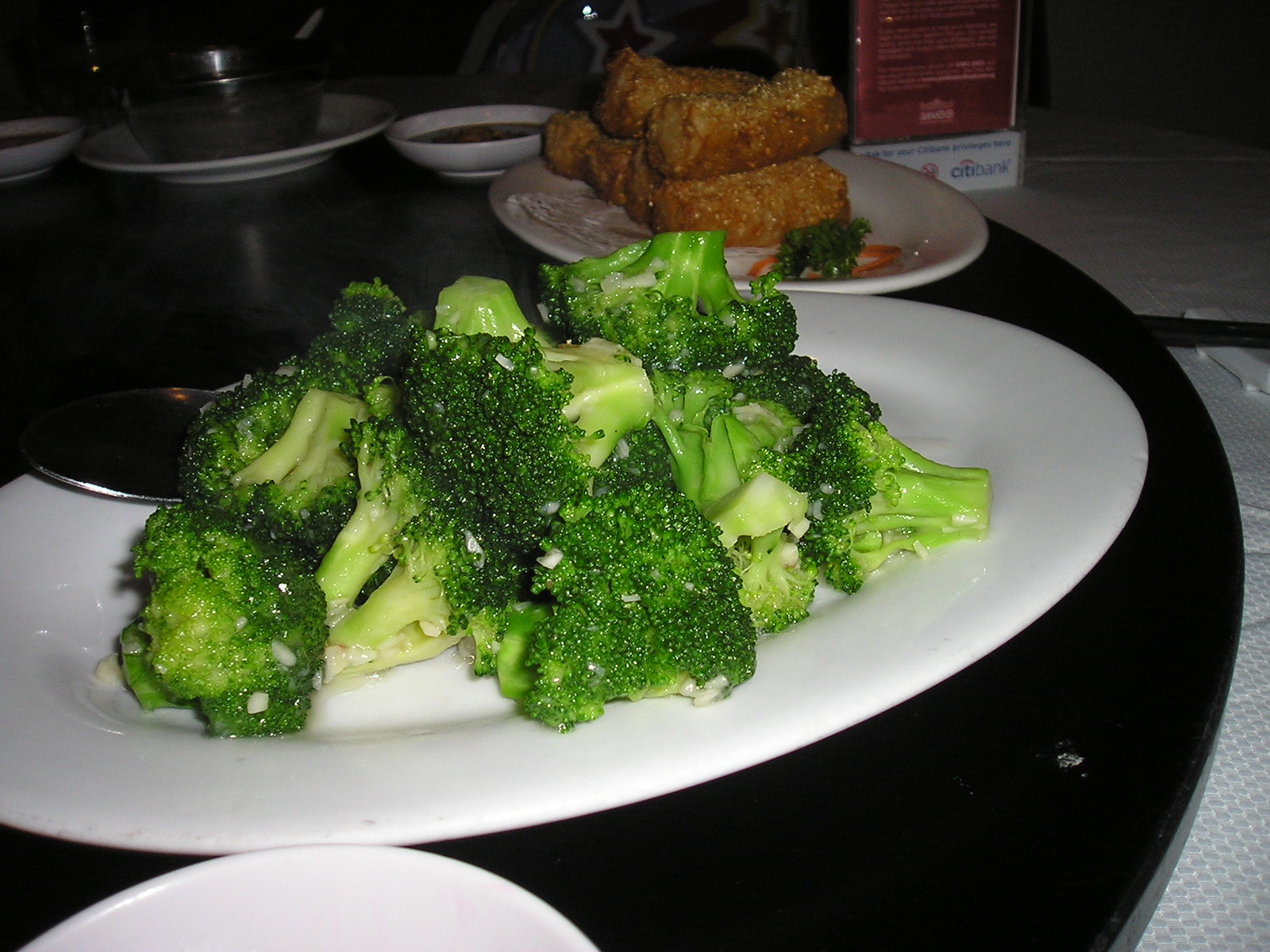The image captures a dimly lit dining setting, likely in a restaurant, featuring a white tablecloth displaying an array of dishes on a large, black, round lazy susan. Central to the composition is a white ceramic plate heaped with vibrant broccoli florets, varying in shades from bright green to dark green and appearing to have been lightly seasoned with a white substance, possibly salt or cheese. Adjacent to this is another white plate holding at least six golden-brown fried egg rolls, with some broccoli scattered around. Further to the right lies a shallow dish containing red sauce. Other white plates are also visible, some with indistinct contents, and there's a subtle hint of a silver spoon among the vegetables. A notable background element is a sign with "Citibank" written in blue text on a white background, capped with a red top band.